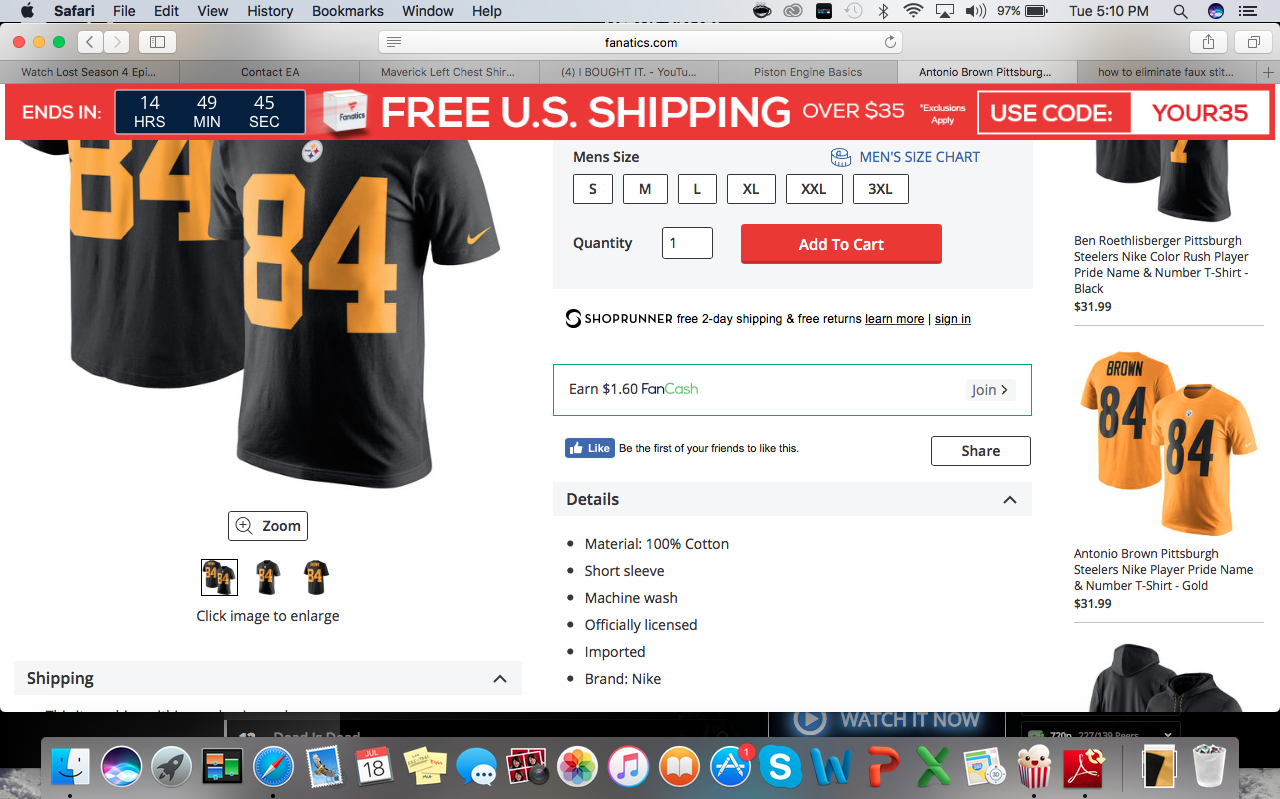The image displays a screenshot of the Fanatics website viewed on a desktop Safari browser on a Mac computer. The URL bar shows "fanatics.com," and a prominent banner at the top advertises free US shipping on orders over $35 with the code "YOURE35." The featured product is a men's Pittsburgh Steelers jersey, predominantly black with a yellow number "84" on both the front and back. The jersey also features the Pittsburgh Steelers logo and a yellow checkmark on the short sleeves. Available men's sizes range from small to 3X large. The quantity selection is set to 1, and the "Add to Cart" button is highlighted in red.

The detailed product description states the following: the material is 100% cotton, it has short sleeves, it is machine washable, officially licensed, imported, and manufactured by Nike. 

A column on the right-hand side of the page suggests additional items for purchase. One suggestion is a black Ben Roethlisberger Pittsburgh Steelers Nike Color Rush Player Pride Name and Number T-Shirt priced at $31.99. Another suggestion is a gold Antonio Brown Pittsburgh Steelers Nike Player Pride Name and Number T-Shirt.